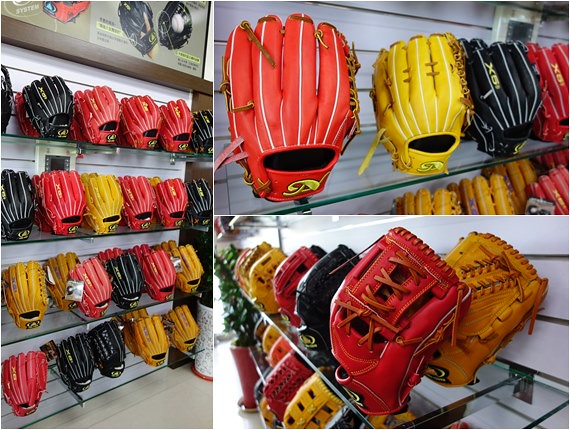The image comprises a collage of three photos depicting a vibrant display of baseball gloves in a sporting goods store. The leftmost photo is a vertical rectangular image showcasing a section of the store with four glass shelves fully stocked with an array of leather baseball gloves. The shelves feature a medley of colors, including red, black, and golden yellow mitts, arranged two deep and six across, suggesting around twenty gloves per shelf. The background gives a glimpse of more sports gear beyond the baseball gloves. 

The top right photograph offers a close-up of one of the glass shelves, highlighting a row of gloves in various colors—red, yellow, black, and another red glove. The black glove bears a logo that might read "X9" or "X6" and some indistinct lettering around the wrist area, which could be "D" or "P". The bottom right image presents a side profile view of the same shelf, giving a different perspective on the neatly arranged mitts. Both close-up photos focus on the intricate details and stitching of the colorful gloves, emphasizing their quality craftsmanship.